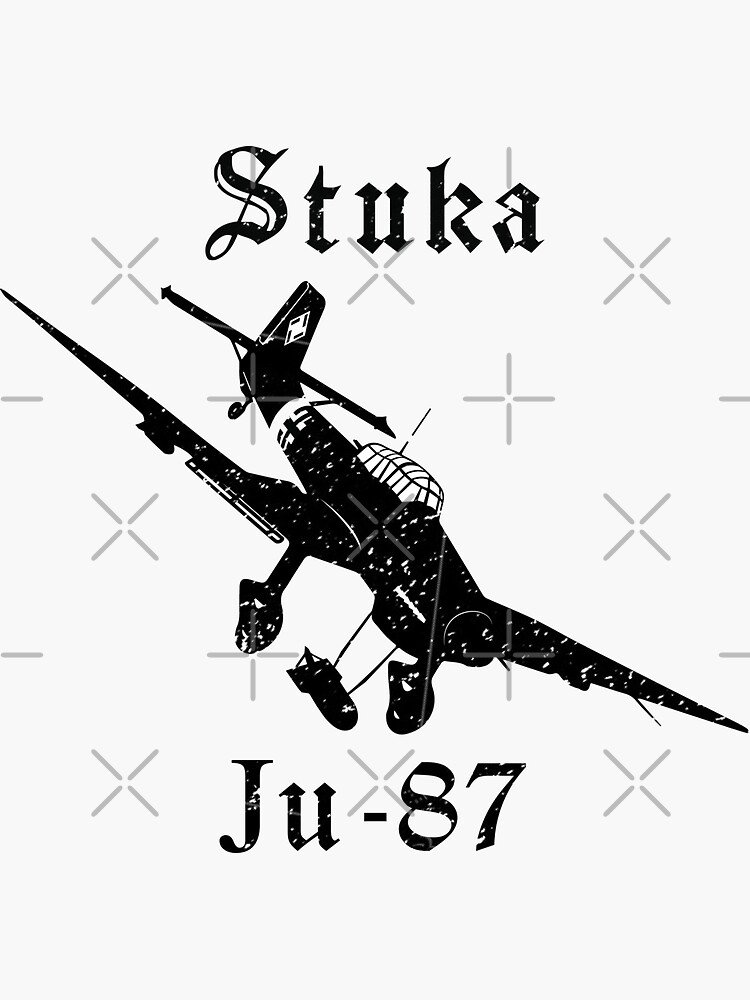The image depicts a vintage, black printed illustration of a single-engine World War II-era airplane, identified as the Stuka JU-87. The words "STUKA Stuka" are prominently displayed at the top, with "JU-87" written at the bottom. The airplane features a distinctive caged dome cockpit and appears to be in a steep dive, showing a bomb suspended beneath its body. The background is white, adorned with light gray X's and pluses acting as a watermark. Notably, the S in "Stuka" is decorative. The plane lacks visible spinning propellers and no pilot is seen in the cockpit. Markings on the tail include a white square with black lines, and further up on the body, there's a cross resembling the British flag. The overall design is rendered in a vintage style, emphasizing a nostalgic aesthetic.